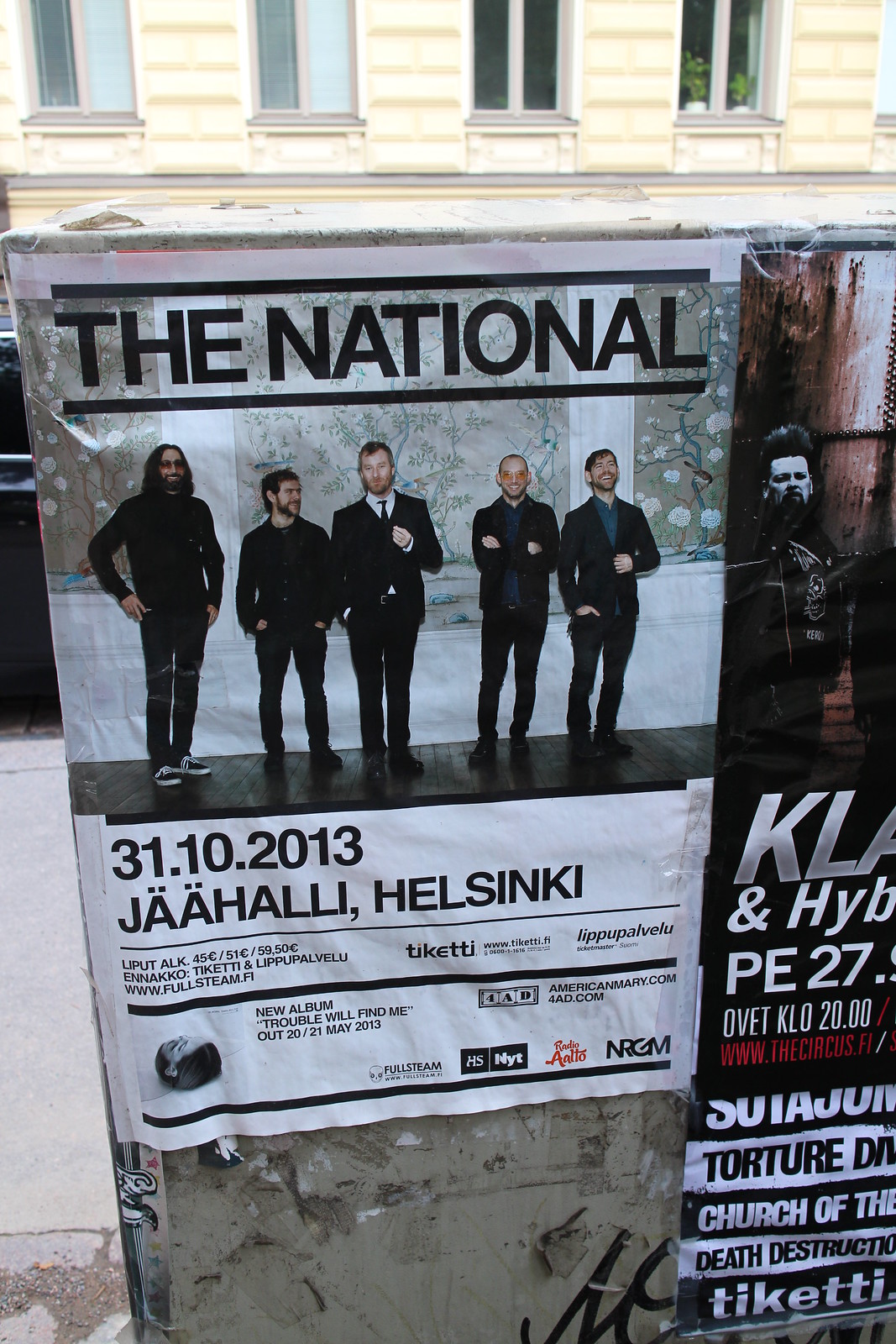The image depicts a slightly cluttered urban scene featuring a poster advertising a concert by the band The National. The poster prominently displays the band name "The National" along with the concert date, "October 31, 2013," and the location in Helsinki. The poster also includes ticket prices and mentions the release of their new album "Trouble Will Find Me" on May 20-21, 2013. Tickets are priced at 45 units of currency, 51 units, and 59.50 units, likely related to seating tiers or early-bird pricing. Additional text points to several URLs, such as www.fullsteam.fi, AmericanMary.com, and 4AD.com, possibly for more information or ticket sales. The poster features an image of five band members, two dressed casually in jeans and sweaters, and three in more formal attire, including one in a white shirt and tie. This poster is affixed to a public fixture, likely a mailbox, surrounded by other flyers and set against an outdoor backdrop where buildings and a sidewalk are visible. To the right of The National’s poster, another advertisement partially visible, possibly for a church event, mentioning themes like destruction and torture.